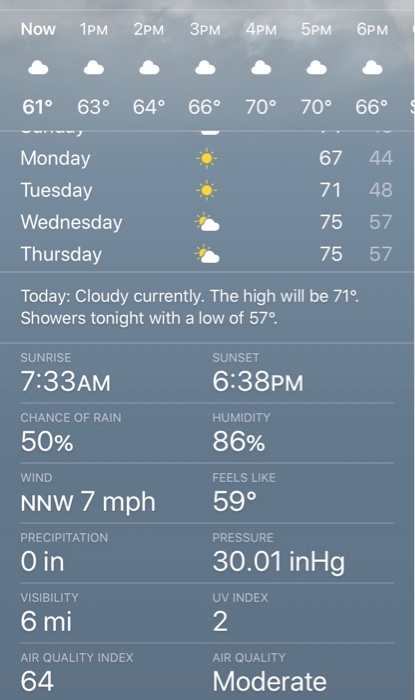This image is a screenshot from a weather website or app with a grayish-blue background resembling the sky. At the top of the screen, thin clouds are faintly visible. Overlaid in white text, the weather report begins with an hourly forecast showing temperatures for the current and next five hours — 1 p.m. to 6 p.m. Each hour is marked with a cloud icon, illustrating cloudy weather. The temperatures listed from left to right are 61°F, 63°F, 64°F, 66°F, 70°F, 70°F, and 66°F.

Below the hourly forecast, there is a vertical daily forecast for the upcoming days. It reads as follows:
- Monday: Sunny, with a high of 67°F and a low of 44°F.
- Tuesday: Sunny, high of 71°F, low of 48°F.
- Wednesday: Partly cloudy, high of 75°F, low of 57°F.
- Thursday: Partly cloudy, high of 75°F, low of 57°F.

Further down, additional information notes that today is currently cloudy with a high of 71°F, and showers are expected tonight with a low of 57°F. 

Supplemental details include:
- Sunrise and sunset times
- Probability of precipitation
- Humidity percentage
- Wind speed and direction
- Information on precipitation, atmospheric pressure, and visibility.